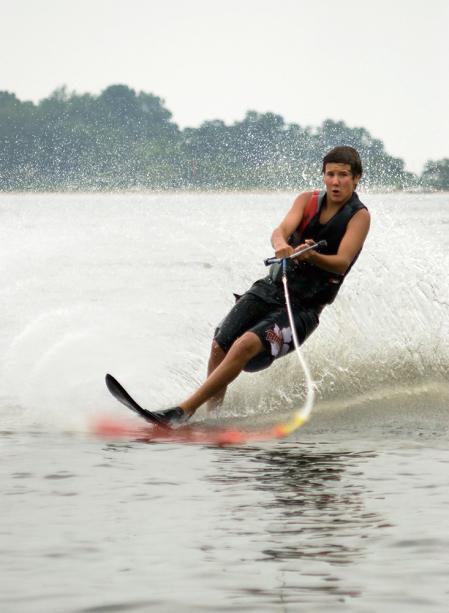In this vivid photograph, a young man, likely in his late teens or early twenties, can be seen engaging in what appears to be wakeboarding or water skiing on a clear, serene lake. Captured from the perspective of the back of a boat, he holds a handle attached to a rope, although the rope's connection to the boat seems puzzlingly submerged in the water. The young man, who has short brown or black hair and is of either Caucasian or Hispanic descent, is firmly gripping the handle with both hands—one hand facing down, the other up—while leaning slightly to his left, causing vibrant splashes of water all around him. He sports a life jacket with black, gray, and red segments over his bare chest and black swim trunks adorned with a white and red logo and a white flower design. His expression is animated, with his mouth open, signaling joy or concentration as he glides across the water's surface. Behind him, the landscape features a grove of trees, completing the picturesque and lively scene.